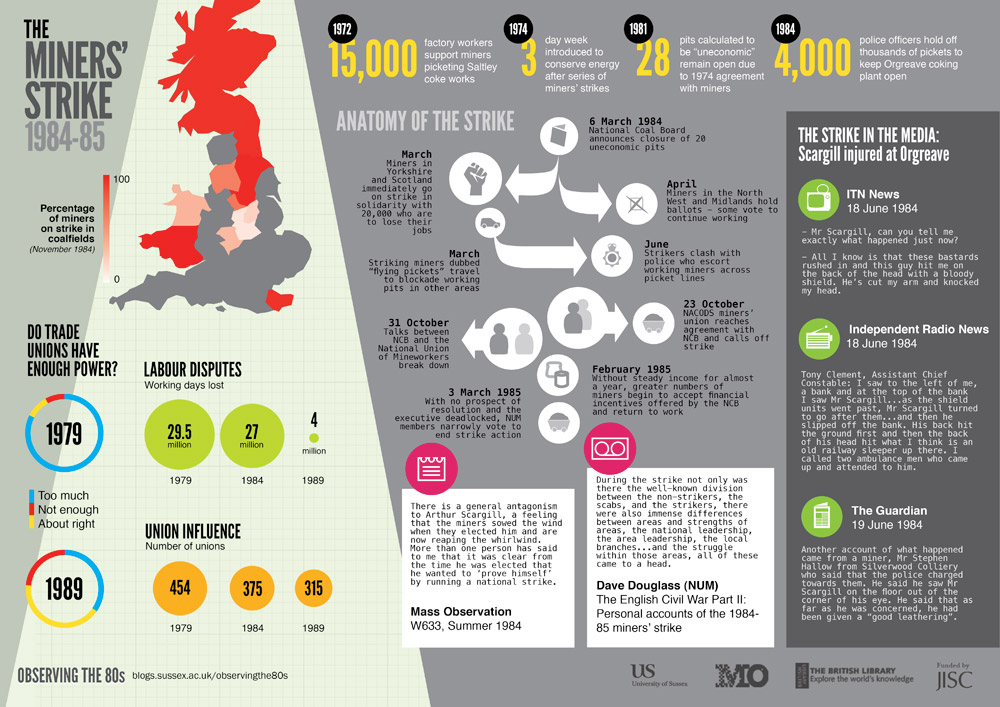This detailed diagram provides a comprehensive overview of the miners' strike in the United Kingdom from 1984 to 1985. The central feature is a map of England, which contextualizes the geographical scope of the strike. Surrounding the map is a detailed timeline that highlights key events and milestones, beginning from 1972, with significant years marked as 1974, 1981, and 1984.

At the top margin, the diagram charts the progression and intensity of the strike over different periods, while also noting significant labor disputes and the corresponding number of working days lost in the years 1979, 1984, and 1989. To provide additional context, the number of trade unions and their influence over time are illustrated, with specific data points showing a decline from 454 unions in 1979, to 375 in 1984, and further down to 315 in 1989.

A thought-provoking question posed within the diagram asks, "Do trade unions have enough power?" This inquiry is visually supported by a chart tracking union influence from 1979 to 1989. In the lower right corner, a section titled "Observing the 80s" encapsulates additional insights, including media coverage of the strike, with a particular note about Arthur Scargill, a key union leader, being injured at Orgreave.

This intricate and multifaceted diagram not only traces the anatomy of the miners' strike but also offers an in-depth look at the broader context of labor union dynamics and the socio-political climate of the 1980s in the UK.